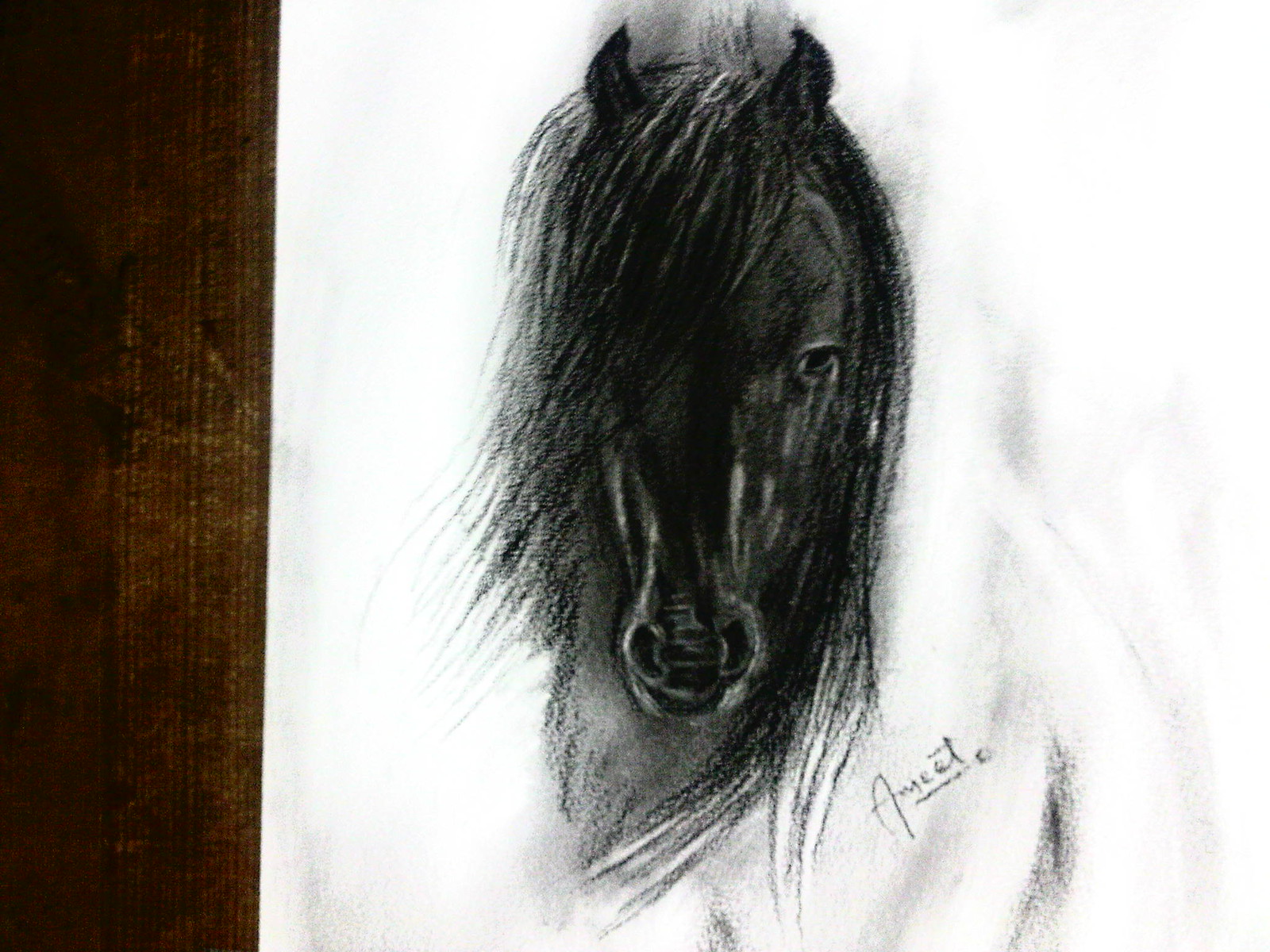This image features a detailed pencil drawing of a black horse's head, meticulously rendered in shades of black, white, and gray. The dark pencil art sits on a stark white background, enhancing the contrast and bringing depth to the illustration. The drawing rests atop a dark brown wooden surface, with the left edge of the wood forming an upward rectangle, suggesting it is part of a table.

The horse's head is beautifully detailed, with a long mane gracefully flowing along the sides of its face. One of the horse's eyes is prominently visible, while the other is concealed by the cascading hair. Notable attention is given to the horse's facial structure, including the finely shaded snout area. The artist, signed as A-M-E-E-T, has skillfully used shading techniques to create a three-dimensional effect, making the illustration captivating and lifelike.